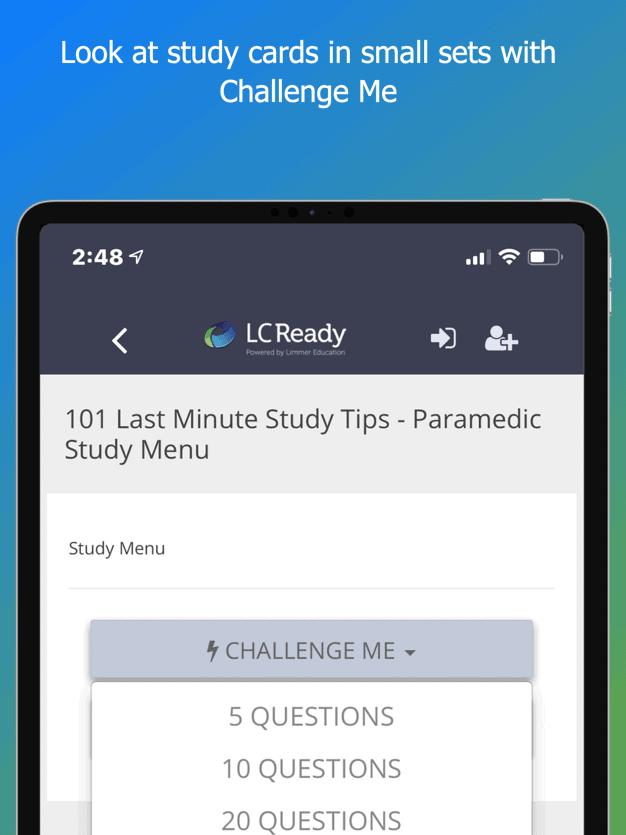The image is a tall rectangular advertisement panel promoting a study tool. The upper section of the image features a blue background with white, centered text that reads: "Look at study cards in small sets with Challenge Me." Beneath the text is an illustration of a smartphone screen, capturing approximately half of its display area.

The smartphone screen shows the status bar at the top with a black border. On the left side, white text displays the numerical figure "248." The right side of the status bar includes white icons indicating cellular connection strength, wireless connectivity, and a half-full battery symbol. Below the status bar, a navigation arrow points to the left, followed by the app name "LC Ready" centered in the middle of the screen. An arrow pointing to the right and an icon representing a person with a plus sign appear next to it.

The main content of the phone screen starts with a gray box containing black text that reads: "101 Last Minute Study Tips. Paramedic Study Menu." Below this, black text on a white background states "Study Menu." Further down, there is another box with a gray background featuring a lightning bolt icon. Alongside this icon, capitalized text reads: "CHALLENGE ME," accompanied by a downward-pointing arrow.

The lower part of the phone screen switches back to a white background with capitalized black text listing options: "5 QUESTIONS, 10 QUESTIONS, 20 QUESTIONS." This marks the end of the visible portion of the smartphone screen within the advertisement.